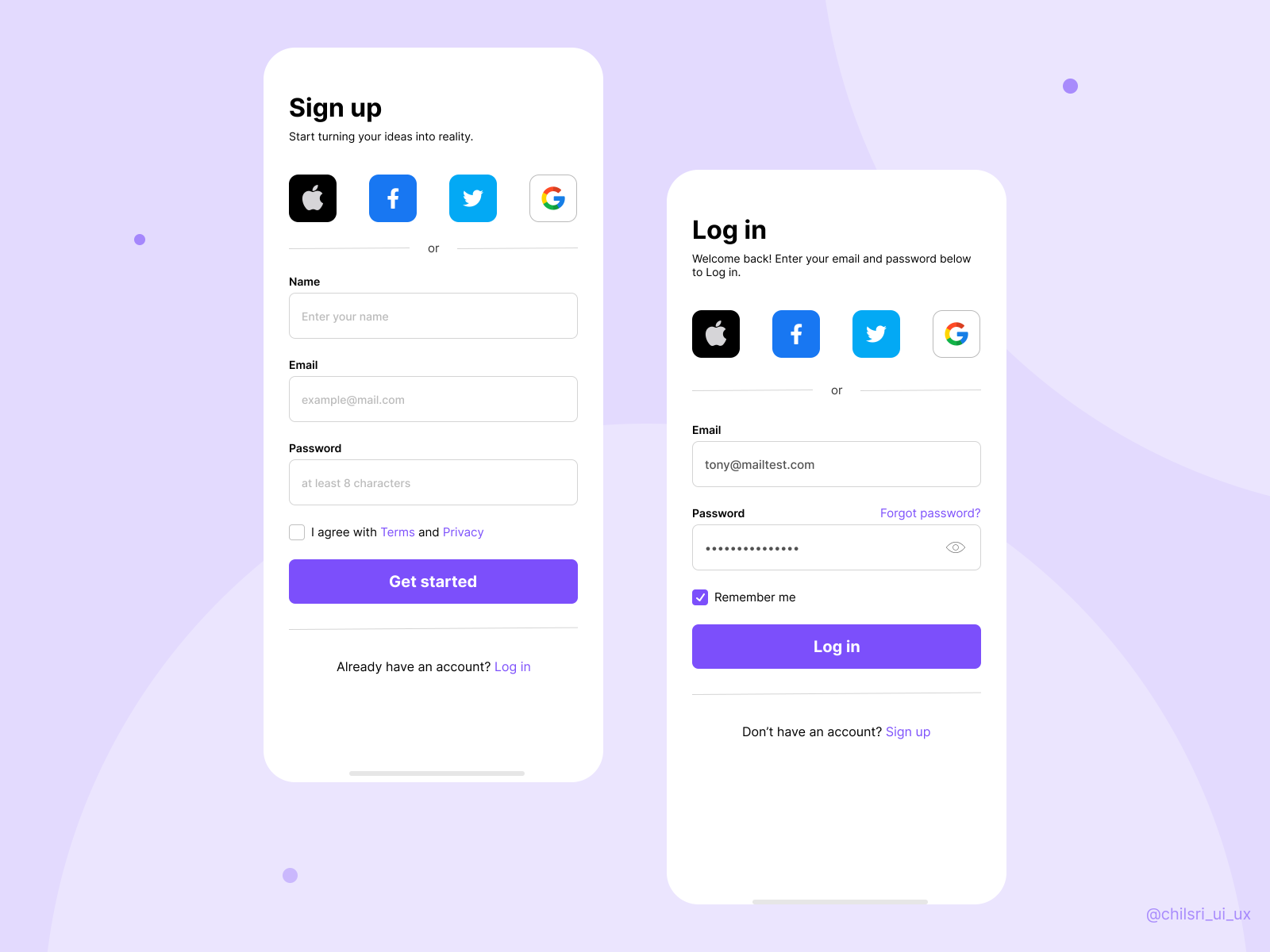The image features two cell phone screens displaying sign-up and log-in options for a service, likely affiliated with Apple, given the visible Apple icon. The first screen invites users to "Sign up" and start turning their ideas into reality. It presents several sign-in options including Apple ID, Facebook, X (formerly Twitter), and Google, and offers the alternative to create a new account by entering a name, email, and password. Users must agree to the terms and privacy policy by checking a box, and can then click the "Get Started" button, highlighted in a purple box. For those who already have an account, a "Log in" option is provided.

The second screen is dedicated to the log-in process, welcoming back existing users with the message "Welcome back." It prompts users to enter their email and password or use the same sign-in options: Apple ID, Facebook, Twitter, and Google. The example shown has the email "Tony@MailTest.com" with the password obscured. There is also an option to "Remember me," which is checked in this instance. The log-in button is clearly visible, alongside a prompt for those who don’t have an account to sign up.

Both screens are set against a pale purple background adorned with circles and small dots, adding a subtle yet stylish design element to the interface.